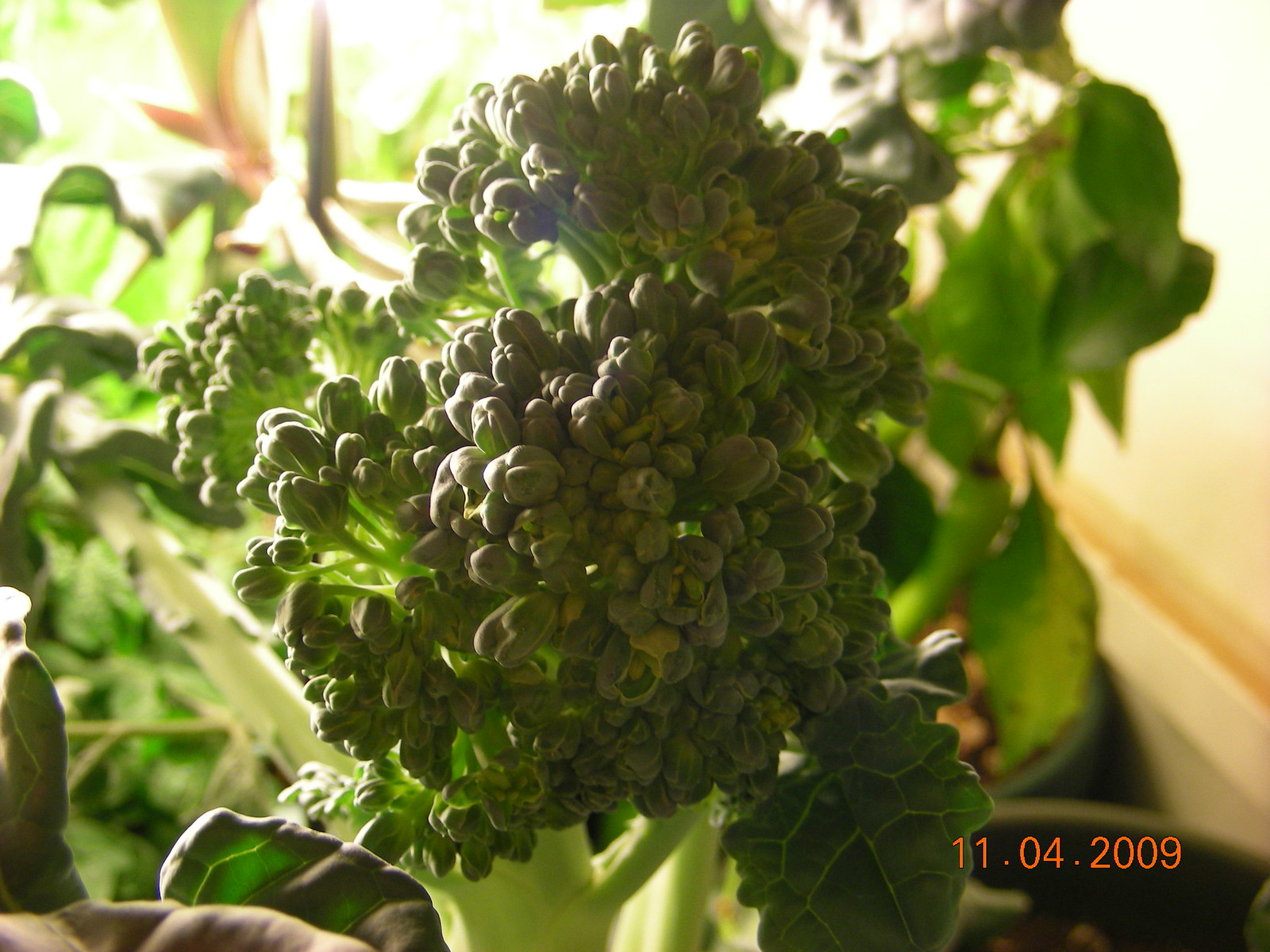This is a color photograph taken indoors, depicting a close-up of a large, green plant with a thick stalk, which extends further into the background, suggesting its considerable size. Dominating the center of the image are multiple small, round green buds on the plant, resembling flowering broccoli or Brussels sprouts. The plant bears a single spiky green leaf, with some leaves appearing wilted and grayish-brown. In the blurred background, several other plants can be seen, including one with tall leaves tinged with yellowish-orange hues and another with droopy, large green leaves. A yellow-colored wall provides a backdrop to the scene. In the bottom right corner of the image, some planters are positioned on the ground, and a date stamp, "11-04-2009," is visible, marking the time the photograph was taken.